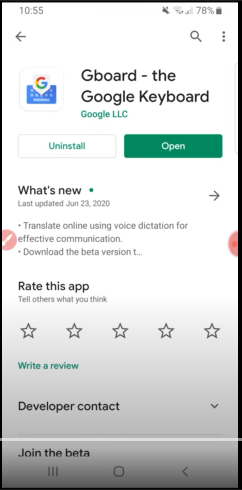Screenshot showcasing the Google Play Store interface for the Gboard app by Google LLC. The top of the screen displays the device's battery level at 78%, with the time being 10:55. The interface includes navigational and functional icons such as a left arrow, a magnifying glass, and three vertical dots.

In the app's details section, Gboard is presented with its icon and developer name, Google LLC, highlighted in green. Below this, there are two prominent buttons: a white rectangle labeled "Uninstall" and a green rectangle labeled "Open." A blue dot next to "What's new" indicates recent updates, with the last update dated June 23, 2020.

Additional options include a right arrow for navigating further, a "Translate" feature suggesting the use of voice dictation for effective communication, and a prompt to download the beta version of the app. Users are encouraged to rate the app with a "Rate this app" section, where five grey stars await user ratings, and a green button labeled "Write a review" invites detailed feedback.

Moreover, there's a section for "Developer contact" expandable via a down arrow, an option to "Join the beta," and navigation icons at the bottom, including three vertical rectangles, a square, and a less than symbol, suggesting the presence of further navigational tools.